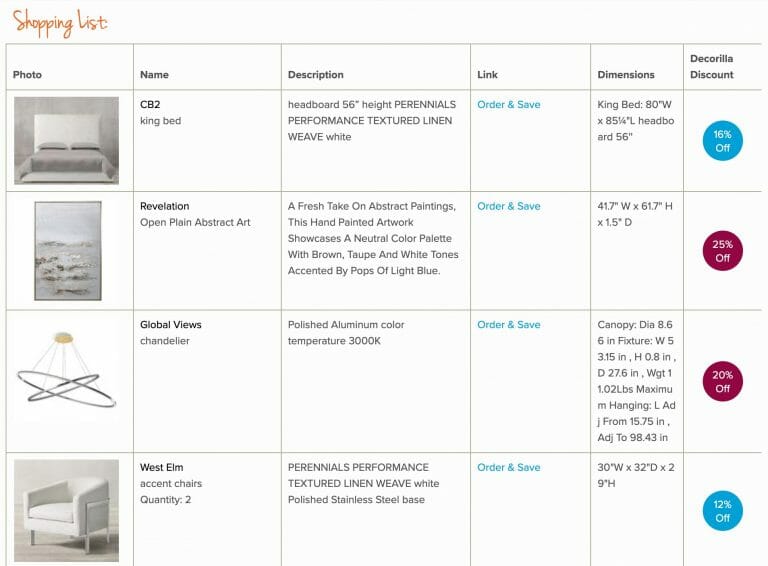This is a detailed caption for the given image:

---

This screenshot features a predominantly white background with "Shopping List" written in orange cursive in the upper left-hand corner. Below this heading, a neatly organized grid with six columns is displayed. The columns are labeled as "Photo," "Name," "Description," "Link," "Dimensions," and "D Corlea Discount," with light orange lines outlining each box. The grid showcases four rows, each containing a photo in the "Photo" column, accompanied by corresponding details across the other columns. Both the "Name" and "Description" texts are written in black. The "Link" column features blue text, specifically the phrase "Order & Save." The "Dimensions" column also contains black text, detailing the size information. The "D Corlea Discount" column comprises circles with discounts, displayed in white text against different colored backgrounds: the top row has a blue circle with "15% Off," the second row has a red circle with "25% Off," the third row has a red circle with "20% Off," and the bottom row has a blue circle with "12% Off."

---

This caption conveys all the relevant details in a clear and organized manner.